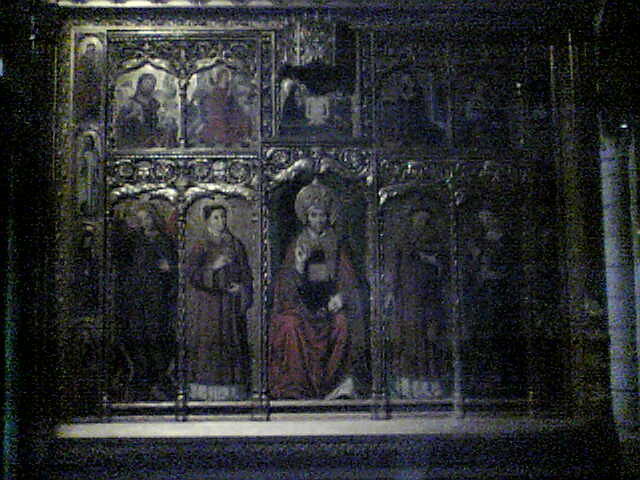The image showcases the interior of a church, focusing on a large, ornate wall adorned with several religious paintings, each encased in an intricate gold frame. At the center of the composition is a seated man, possibly a religious figure or priest, dressed in elaborate long red robes and featuring a gold halo around his head. He has a beard and raises one hand with a finger pointing upwards. Flanking him are two figures on each side, all wearing robes, possibly monks, also involved in a religious scene. Above these central figures are smaller framed images, depicting additional robe-clad individuals, some of whom also have gold halos. A light subtly illuminates the upper left portion of the wall, adding depth to the dark and somewhat grainy overall appearance of the image. The gold framing and ornate detailing suggest a traditional and solemn religious setting.